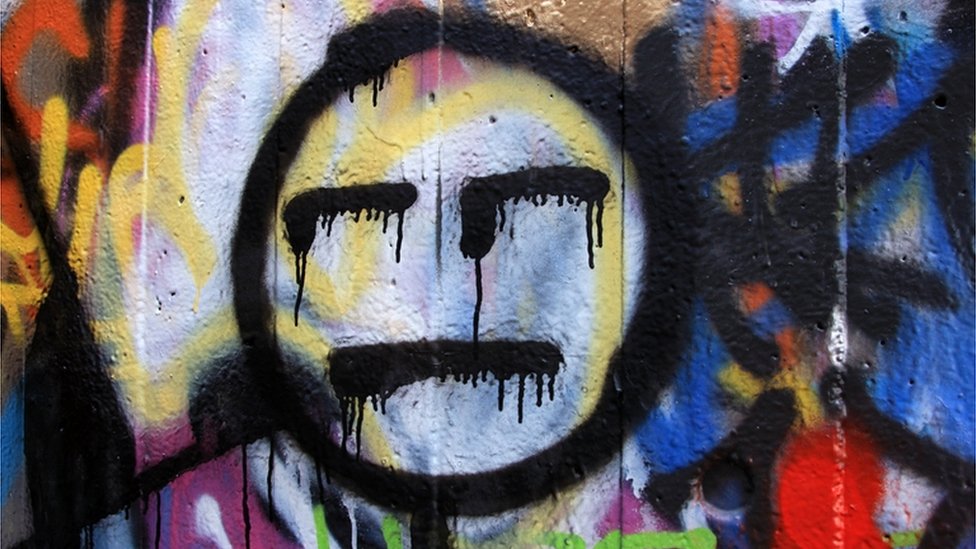The image depicts a vibrant piece of graffiti art on a concrete wall. The wall, composed of segmented boards with visible vertical lines, serves as the canvas for this colorful artwork. The graffiti features a central black circle that depicts a face with two black eyebrows and a straight-lined mouth, both of which have paint dripping down vertically. The interior of the face is painted with white and accented with yellow curves. Surrounding the face, the background bursts with a kaleidoscope of colors including yellow, orange, blue, red, purple, and green, creating a lively contrast against the grey, concrete texture of the wall. The overall effect is both chaotic and meticulously planned, blending the rawness of street art with a touch of abstract expressionism.